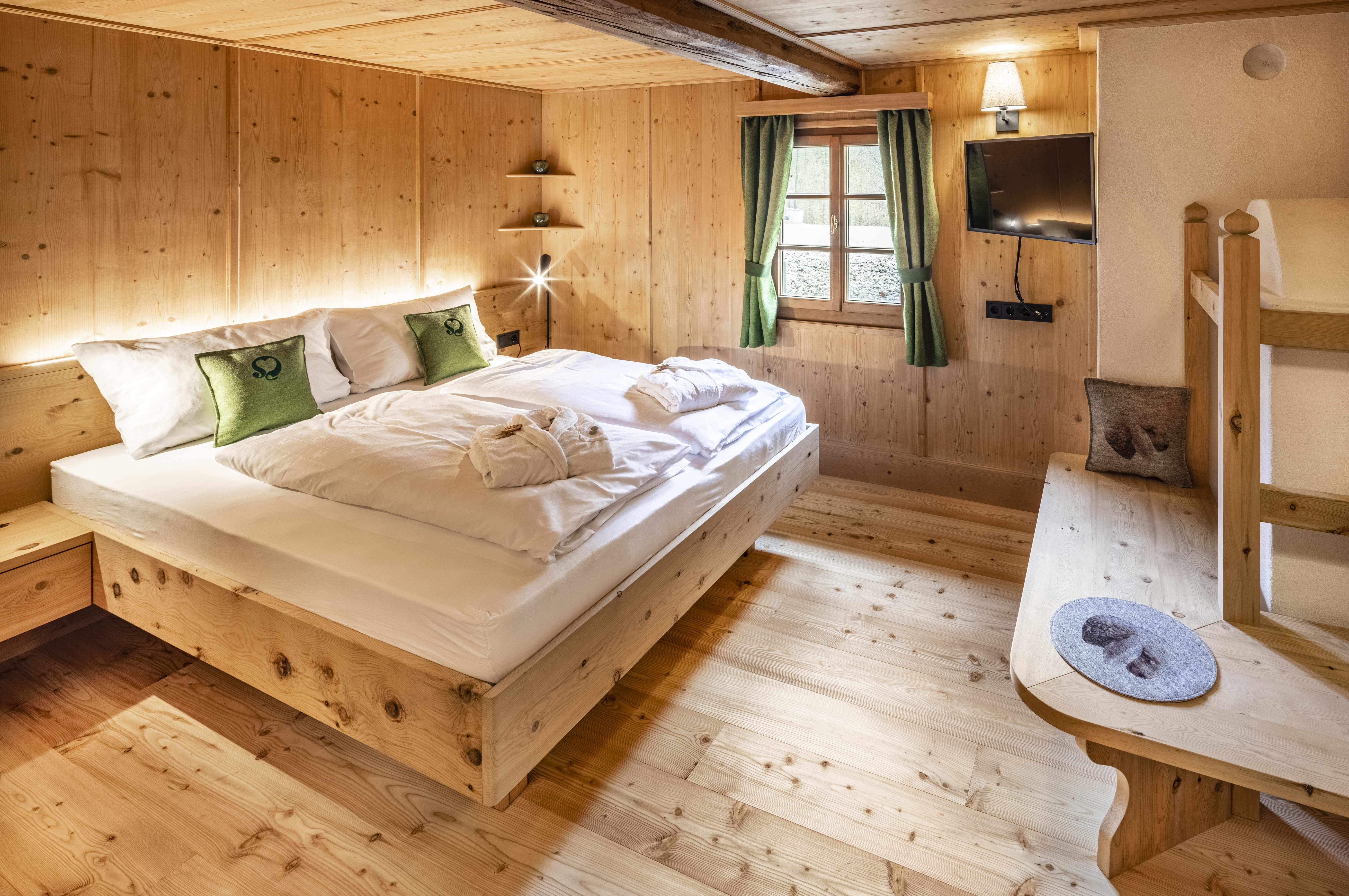The image depicts a modern log cabin bedroom that exudes a cozy, rustic charm. Dominated by a consistent two-by-four wooden finish that extends from the platform bed to the walls and flooring, the room features a king-sized bed adorned with crisp white sheets, two white pillows, and two smaller green accent pillows. Atop the bed rest two neatly folded white robes, suggesting a welcoming touch characteristic of a bed-and-breakfast or an Airbnb. Across from the bed stands a piece of furniture, possibly a bench, constructed from the same light-colored wood as the bed frame and other elements in the room—including built-in shelving in the corner. A flat-screen TV is mounted on the wall in one corner, with a lamp positioned just above it. The window is dressed with green curtains, and a glimpse outside reveals a serene, green landscape. The simplistic, unstained wooden decor is subtly enhanced by LED lights behind the bed's headboard, adding a touch of modernity to the rustic ambiance.